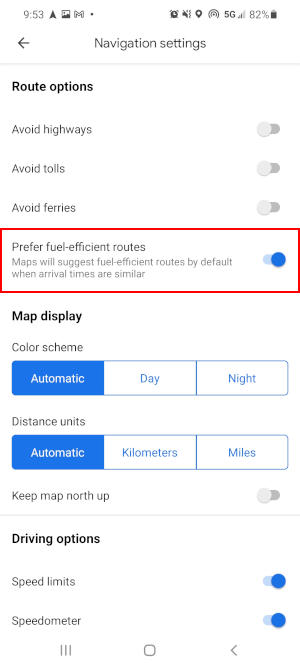This screenshot displays the navigation settings interface. At the top, "Route Options" is prominently highlighted. Below, users can choose to avoid highways, tolls, or ferries via individual toggle switches, all of which are currently turned off. Further down, there's an option labeled "Prefer fuel-efficient routes," which is activated, and indicated by an orange rectangle; this ensures that Maps will suggest fuel-efficient routes by default when the arrival times are similar.

Following this, "Map Display" is also bolded. The first setting here is the color scheme, illustrated by three side-by-side blocks. The "Automatic" option is selected and marked in blue, while the alternative "Day" and "Night" options remain unselected. Next, the distance units setting is shown, offering automatic, kilometers, or miles, with "Automatic" currently chosen. Another setting in this section is "Keep map north up," which is an unselected toggle switch.

Finally, under the "Driving Options" heading, both "Speed Limits" and "Speedometer" settings are toggled on, ensuring these features are enabled during navigation.